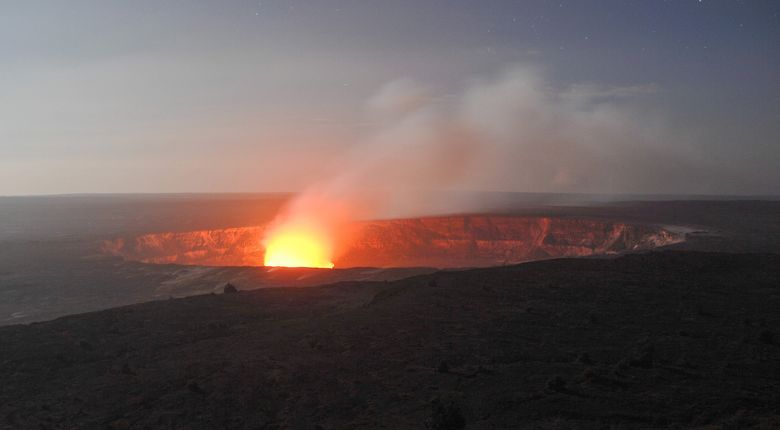The image depicts an outdoor night-time scene, centered around a large crater or cavernous opening in the ground, which bears a striking resemblance to a volcanic vent. Dominating the left side of this opening is a prominent, glowing fireball, casting a bright yellow light that illuminates the crater, giving it a reddish hue. This intense light source is surrounded by dense smoke, billowing upward and obscuring parts of the sky. The surrounding land appears flat and dark, covered in ash or soot, with minimal to no vegetation visible. The sky above the darkened landscape is predominantly overcast and smoky, with a small clear patch in the top right corner revealing a touch of blue haziness, suggesting the presence of thick cloud cover or lingering smoke. The overall atmosphere is dim, the only significant illumination emanating from the fiery glow within the crater.